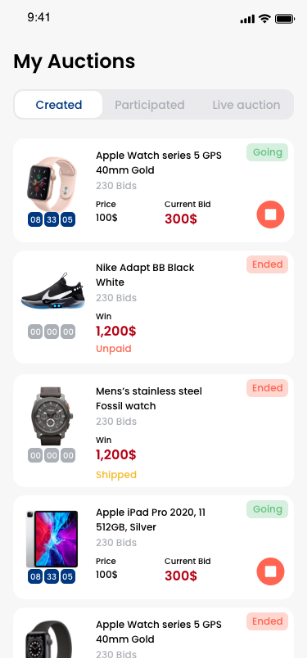This detailed screenshot of a mobile auction application resembles an eBay-style platform, yet distinct in its design. Displayed on a user's phone, the top left corner shows the time "9:41" in black, while the top right indicates a strong cell phone connection, active Wi-Fi, and a fully charged battery, all displayed against a gray background. 

The main display area highlights a white background featuring the user's auction details. At the top, the larger font "My Auctions" is prominently displayed in black. Below it, a white button labeled "Created" in blue stands out, flanked by grayed-out options "Participated" and "Live Auction."

The screen showcases five active and past auctions, each detailing an image of the item, the auction duration, the item's title, its original price, and the current bid amount. The top auction is for an "Apple Watch Series 5 GPS 40mm Gold," still active. Following this is a "Nike Adapt BB Black White" with 230 bids, showing a winning bid of $1,200, yet unpaid. Next, a "Men's Stainless Steel Fossil Watch" also with 230 bids, lists the winning bid of $1,200 as paid and shipped. Farther down, an ongoing auction for an "Apple iPad Pro 2020 11, 512GB Silver" shows the original price of $100 and a current bid of $300. 

The last visible auction is again for an "Apple Watch Series 5 GPS 40mm Gold." Although the bid has ended, detailed information is obscured as it is cut off from view. Each item is accompanied by clear and attractive images within a clean, user-friendly interface.